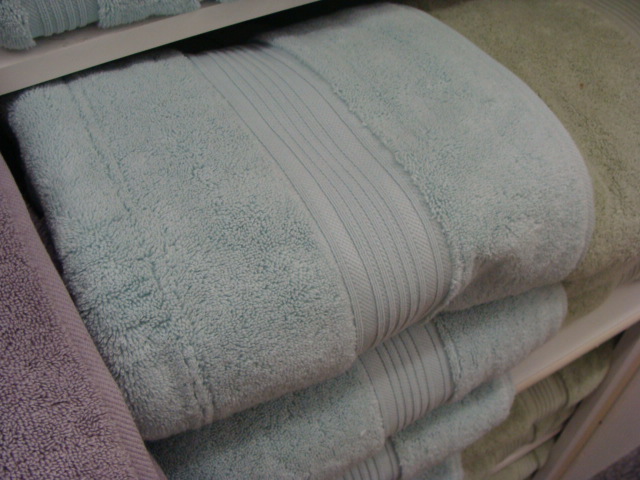This close-up photograph, taken inside a textile or homeware store, showcases neatly folded bath towels organized on cream-white shelves. In the foreground, a stack of light aqua blue towels with a ribbed banding in the middle extends vertically downwards. To the right of the blue towels, there is a stack of identical olive green towels. The image reveals multiple levels of shelving: the bottom left corner features a light maroon towel partially cut off, while above and below these blue and green stacks are more of the same towels placed meticulously. The perspective suggests the photo was taken at a 45-degree angle, possibly with a smartphone, capturing the orderly arrangement from a first-person view. The upper left of the image shows a partial glimpse of another cream-white shelf above, hinting at additional blue towels just out of full view. Overall, the arrangement exudes tidiness and highlights the textured design in the center of each towel, emphasizing their fluffy cotton material.